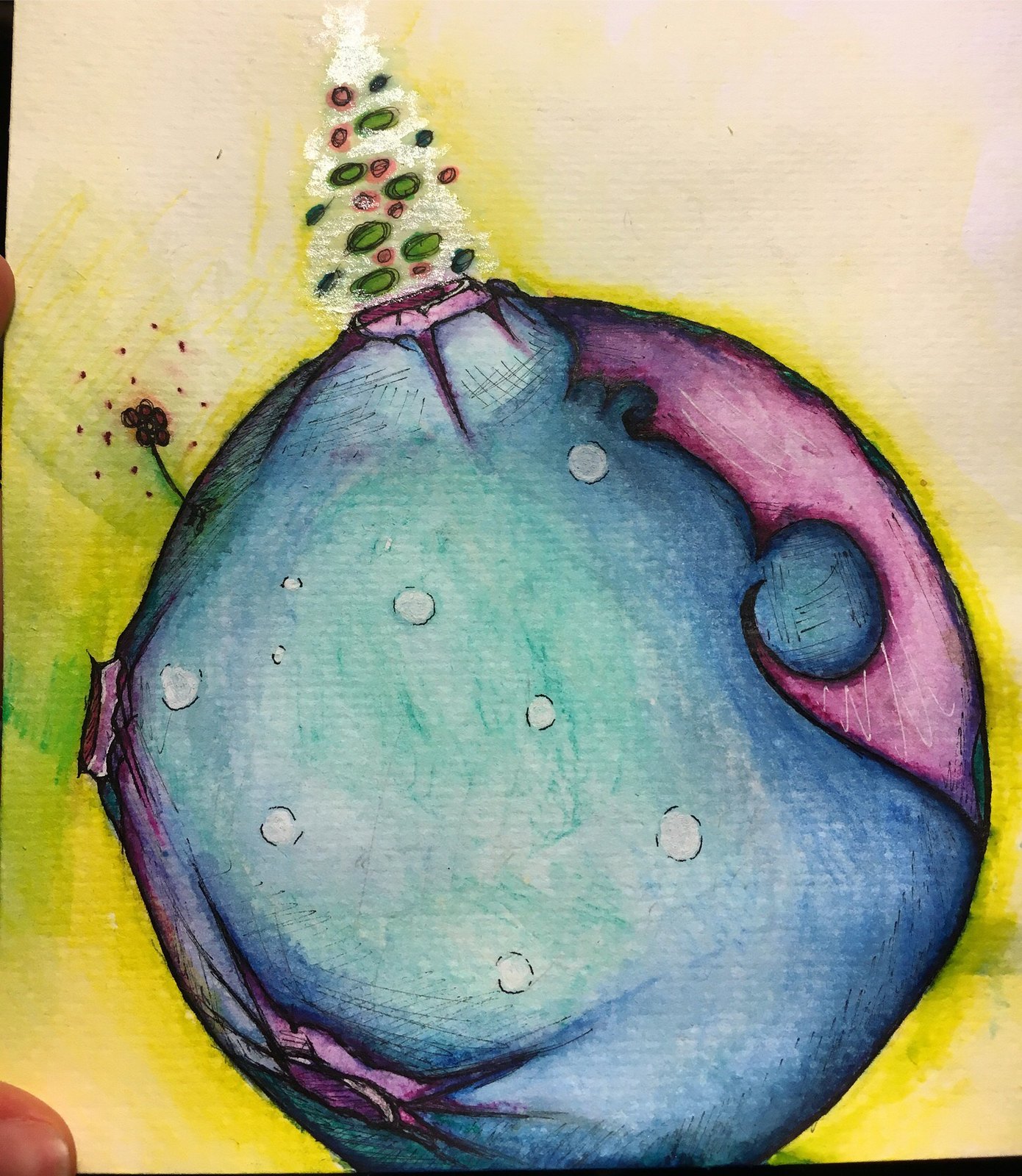The image is a detailed and surreal drawing of a Christmas ornament created with a combination of crayon and watercolor techniques. The ornament, primarily circular in shape, features hues of blue in the front and purple towards the back, with various white spots and one side appearing cracked or peeled away. This peeling portion forms into a Christmas tree, adorned with red and green bulbs that resemble jewels.

At the top of the ornament, angled slightly to the right, is a white Christmas tree decorated with red and green dots, mimicking the look of lights. Behind this ornament, to the left, is a whimsical, wish-like flower with five red petals and a visible stalk, accompanied by numerous small red dots.

The background of the image transitions from a peach color at the top to a yellow haze with streaks of blue, giving it a dreamy atmosphere. The entire drawing is outlined in yellow, adding to its surreal quality. In the bottom right corner of the image, you can see the tip of a person's thumb holding up the paper, and parts of their fingers are visible in the top left corner as well, along with some black areas in both corners. The intricate combination of colors and elements makes this artwork both festive and fantastical.